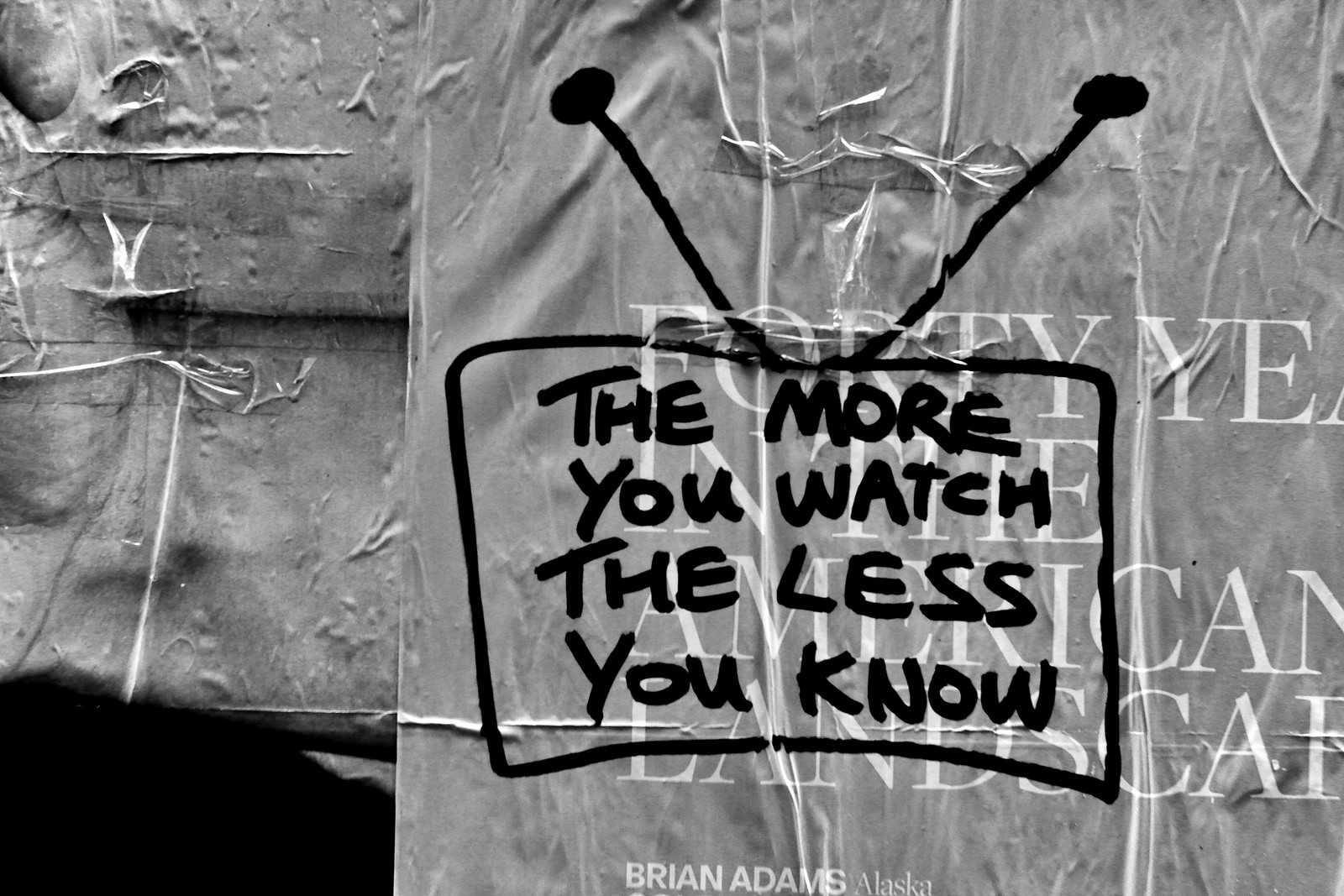The image depicts a black outline of a TV, drawn with a black magic marker, complete with two antennas extending upwards. Inside the TV, the message "The more you watch, the less you know" is inscribed in the same black marker. The TV drawing is superimposed over a background that appears light gray with a texture resembling white torn threads. Behind the TV, there are white, capitalized words that are mostly obscured by the outline. The background itself looks like crushed or shrink-wrapped plastic. At the bottom of the image, the text reads "40 years in the American landscape by Brian Adams, Alaska," marked clearly, with an additional notation of the year 1993, contrasting with the current year 2023. The image seems to mix themes of media consumption and its impact on knowledge.